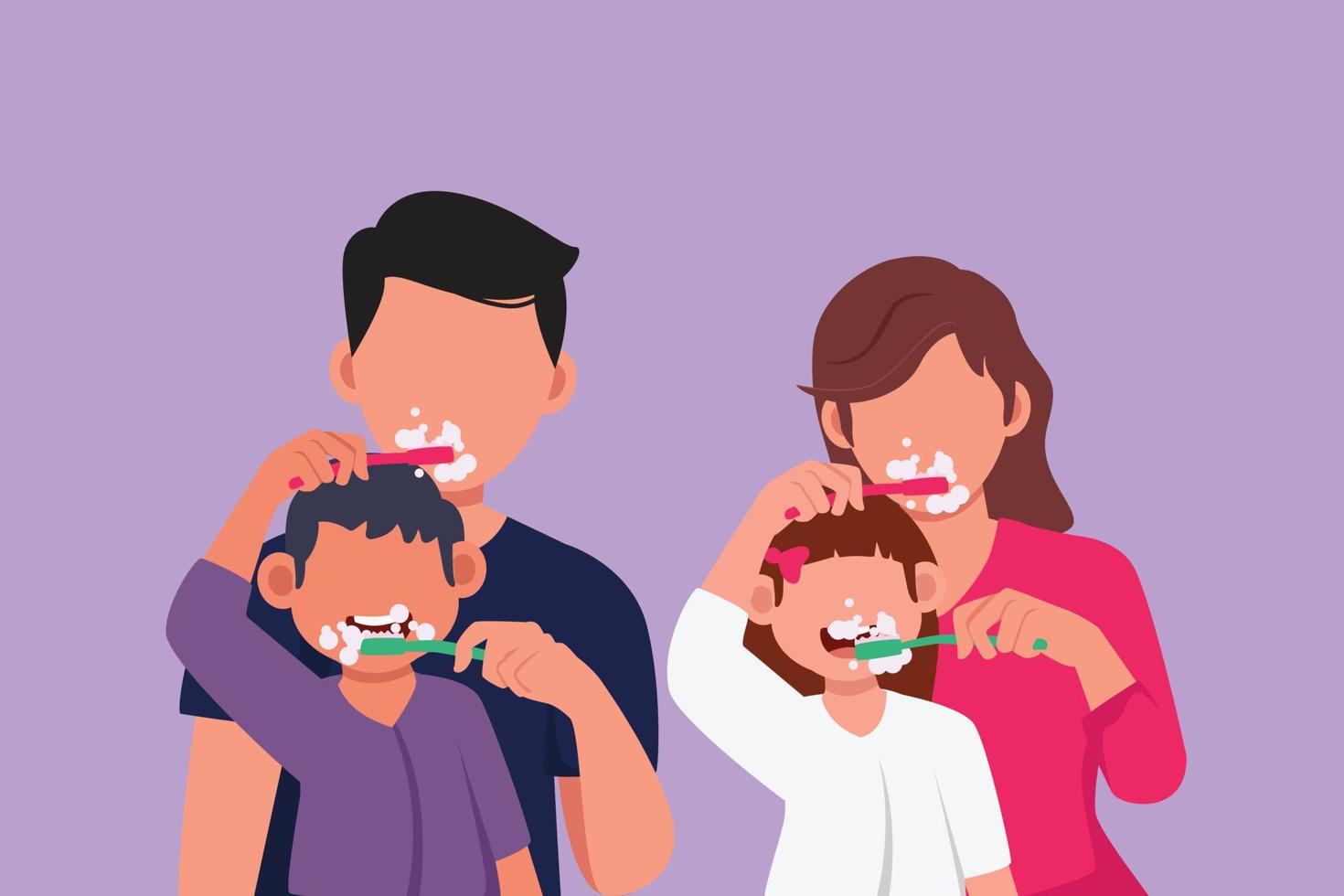The image is a rectangular, computer-generated art piece, characterized by its predominantly light lilac purple background. At the center, four faceless figures (two adults and two children) are engaged in an activity, likely depicting a family brushing their teeth. The figures don't have detailed facial features, but their mouths are illustrated.

On the left side, a man with black hair and a navy blue t-shirt holds a green toothbrush in his left hand, brushing the teeth of a little boy with black hair and a purple shirt. The boy, in return, is using a red toothbrush on the man's mouth, and both their faces are smudged with foamy white toothpaste. Both characters have visible toothbrushes and toothpaste.

On the right side, a woman with long brown hair in a pink shirt (or dress) holds a green toothbrush in her left hand and is brushing the teeth of a little girl who has long brown hair adorned with a pink bow and is wearing a white shirt. The little girl is using a pink toothbrush to brush the woman's teeth. Similar to the left pair, there is a visible toothpaste foam around both their mouths, emphasizing the brushing action.

All figures have an off-beige skin tone, and the overall scene is imbued with a playful, whimsical quality due to the depiction of mutual tooth brushing and the use of vibrant, contrasting colors on their outfits and toothbrushes.